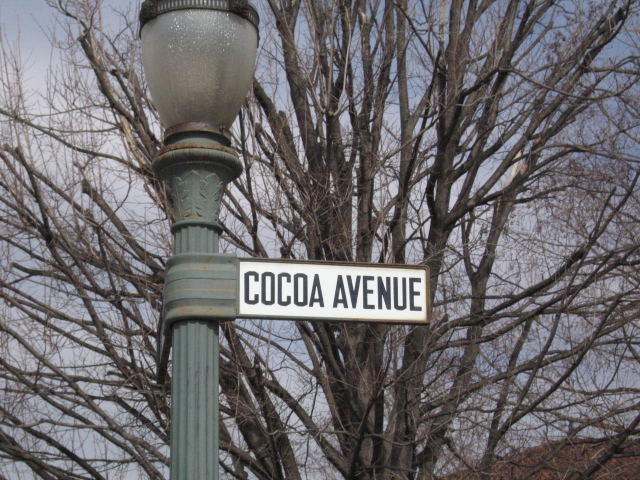In the photograph, an antique street lamp stands prominently in the foreground, evoking the charm of the early 19th century. The lamp, likely crafted from metal, features a glass globe encased by a decorative metal cap and adorned with ornate tiers beneath the globe where the bulbs would be lit. Extending from the street lamp is a street sign that reads "Cocoa Avenue." Behind this scene, a large, leafless tree stretches its intricate network of branches against a backdrop of overcast blue sky, signaling the dormant beauty of winter.